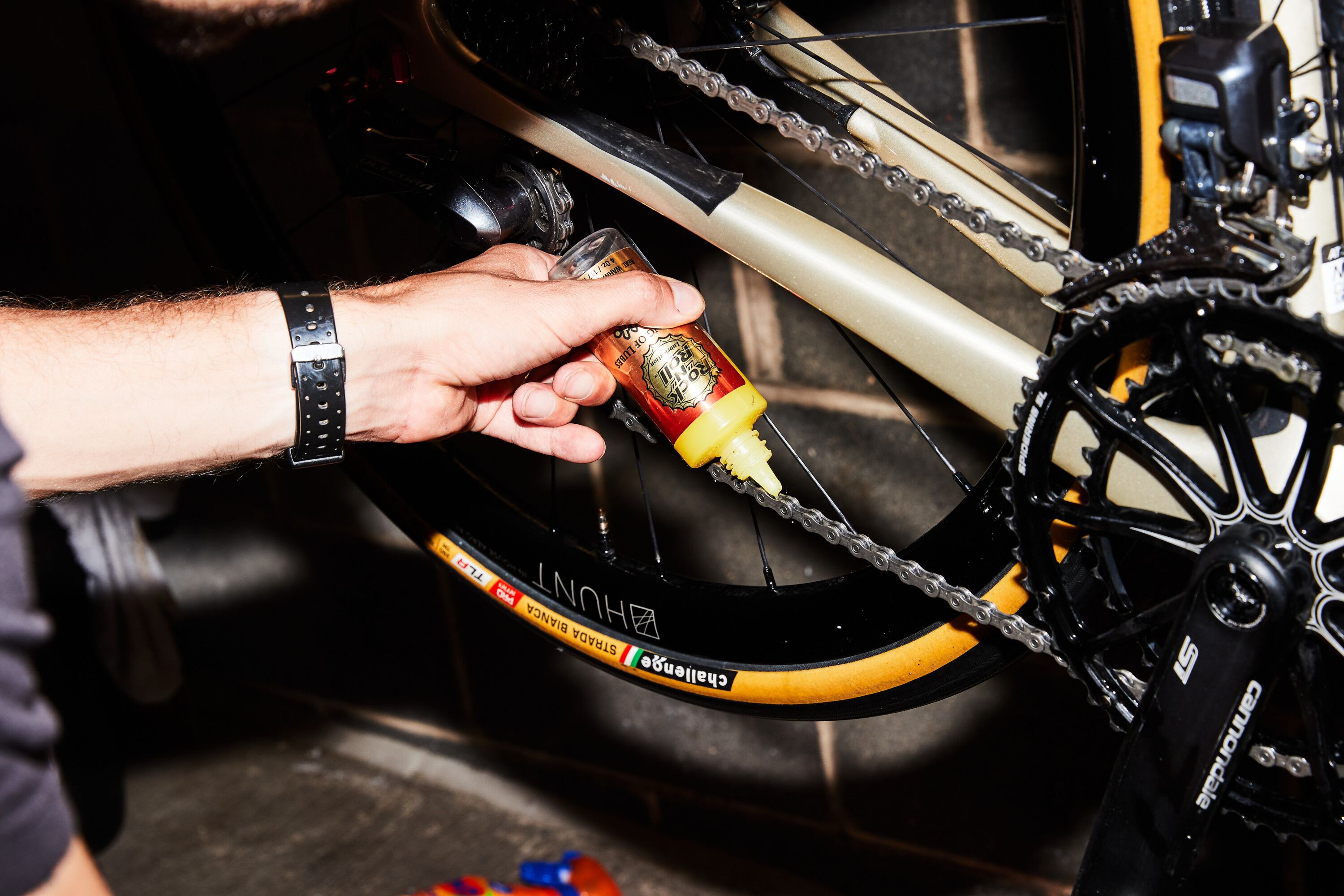In the photograph, a person is oiling the silver chain of a bicycle that is mounted on a rack. They are using a clear plastic bottle filled with a yellowish liquid lubricant, which has a pointed top and a label reading "Rock and Roll Lubrication." The individual is wearing a short-sleeved, dark blue shirt and a black wristbanded watch. The bicycle features a tannish-gray frame with black pedals that have shoe clasps and a cog wheel attached to the chain. The bike has black tires adorned with large orange stripes on the sides and the word “Challenge” visible on the tire rims. The black crank arm at the pedal includes white writing that states the brand "Cannondale." The thin bike tires and the additional sprocket detail suggest that it is a road bike.